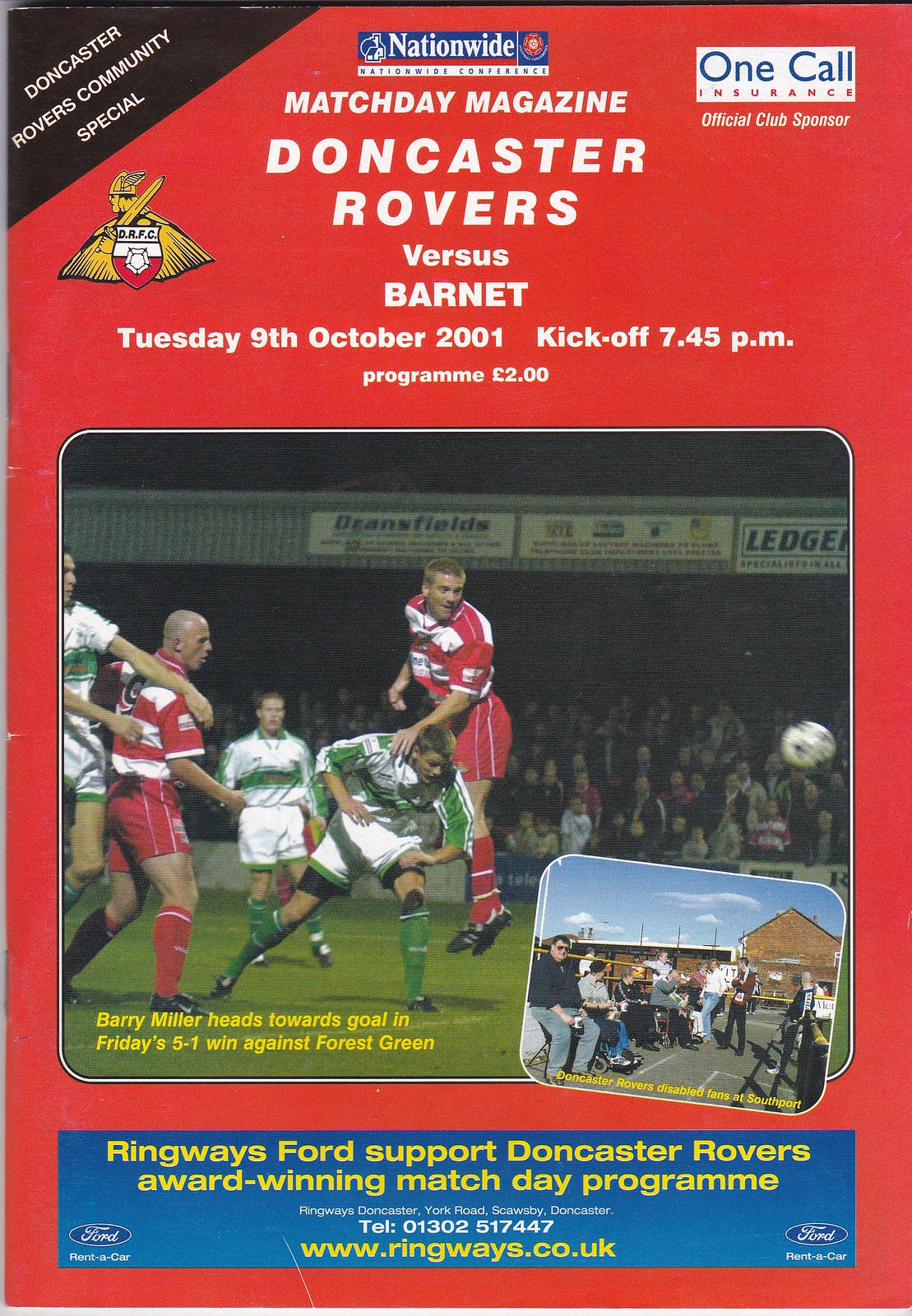The advertisement page features a vivid red background with comprehensive details about the Doncaster Rovers Community Special Nationwide Conference Match Day Magazine. At the top left corner, a black triangle with white text reads "Doncaster Rovers Community Special," while the top section of the page advertises Nationwide. Adjacent on the right, the OneCall Insurance logo appears with the note "Official Club Sponsor." The central portion of the page specifies the event: "Match Day Magazine, Doncaster Rovers vs. Barnet, Tuesday, 9th October 2001, Kickoff 7.45 PM, Program £2."

Below this, a prominent photo captures the dynamic action of the match. It shows a footballer in a red and white kit jumping, supported by a player in a green and white kit, with additional players in matching uniforms on the left and a crowd in the bleachers in the background. The caption beneath the image states, "Barry Miller heads towards the goal in Friday's 5-1 win against Forest Green."

Adjacent to the main image is a smaller inset photo depicting Doncaster Rovers' disabled fans at Southport. At the bottom, a blue banner features a Ford Rent-A-Car advertisement, including the text: "Ringways Ford support Doncaster Rovers award-winning match day program," along with the address and contact details, "York Road, Scosby, Doncaster, Telephone 01302 517447" and the website "www.ringways.co.uk."